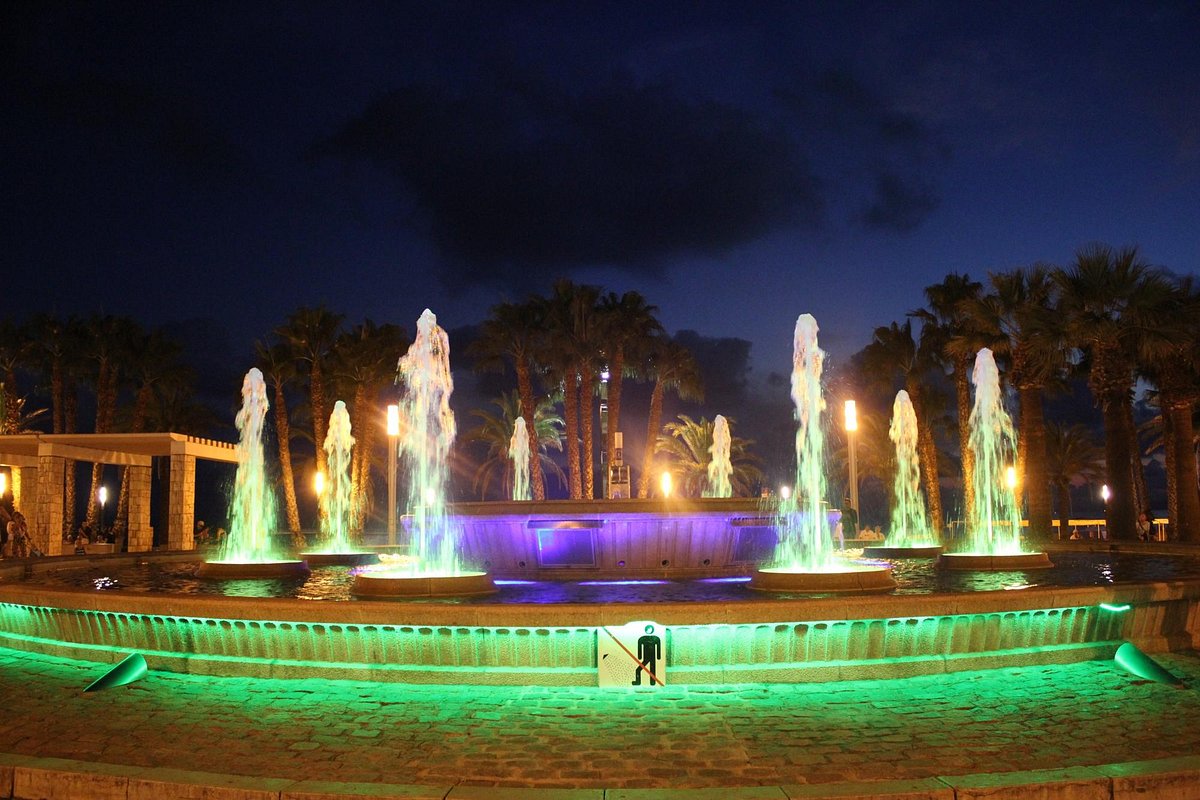This image captures an outdoor nighttime scene centered around an illuminated fountain. The fountain, which has a greenish glow, stands prominently in the middle of a circular platform, encircled by nine smaller water spouts. Surrounding the fountain are several palm trees, suggesting a tropical locale. In the background, a navy blue sky filled with heavy, dark clouds and a hint of stars sets a dramatic scene. At the base of the fountain, there's a white sign depicting a black figure with a red diagonal mark, indicating that people are not allowed in the water. Adjacent to the fountain, to the left, sits a small brick structure, adding to the architectural interest. The overall ambiance is enhanced by the colorful lights reflecting in the water, casting hues of green, purple, white, yellow, and blue throughout the scene.